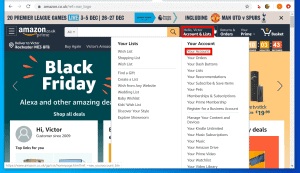The image displays a webpage with a typical browser interface. At the very top, the browser address bar shows navigational icons - a left arrow, a muted right arrow, and a refresh button. The web address is centered within the address bar. To the right of the address bar, there is a star icon followed by additional icons.

The webpage background features a gradient transitioning from a brighter light blue on the left to a darker blue on the right, especially near the bottom.

At the top of the displayed page content, there’s a somewhat blurry headline mentioning "20 Premier League games," followed by the dates "3 to 5 December" and "25 or 26 27 December."

Beneath this text, the word "Amazon" is prominently displayed alongside a search bar. Positioned towards the right side of the screen, a section outlined with a red border contains some text. Adjacent to this, a "Black Friday" graphic with a darker jade blue-green background is visible.

Below this, a drop-down menu banner displays options such as "Your List" and "Your Account," with parts of this banner also highlighted with a red border.